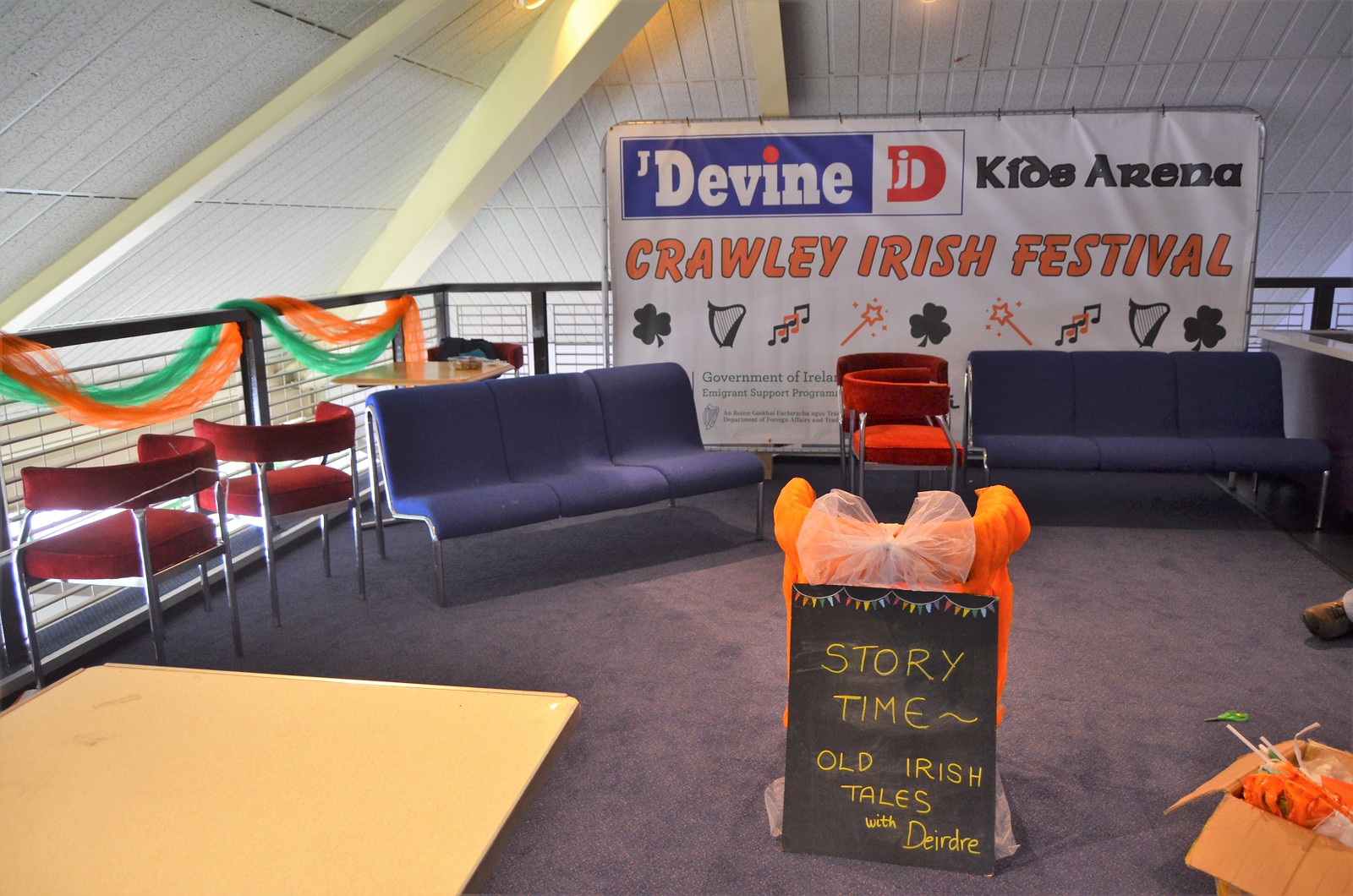This photograph captures an upper-floor indoor setting, showcasing the venue for a Storytime event at the Crawley Irish Festival. The ceiling features a white roof accented with off-white beams, visible across the space. Enclosing the area is a black perimeter fence designed to prevent falls to a lower level. The floor is furnished with various chairs and couches; single chairs are red and the couches are a medium blue, all built on aluminum frames. Prominently displayed in the foreground is a blackboard leaning against an orange structure, announcing "Storytime Old Irish Tales with Deidre." In the background, another sign reads "Divine DJ, Klo Arena, Crawley Irish Festival." This banner is set on a white tarp with orange lettering, while the word "Divine" is highlighted in white letters within a blue box, featuring a distinct blue dot above the 'i'. Overall, the photograph effectively presents the cozy, festive atmosphere of this storytelling event within the greater Crawley Irish Festival.